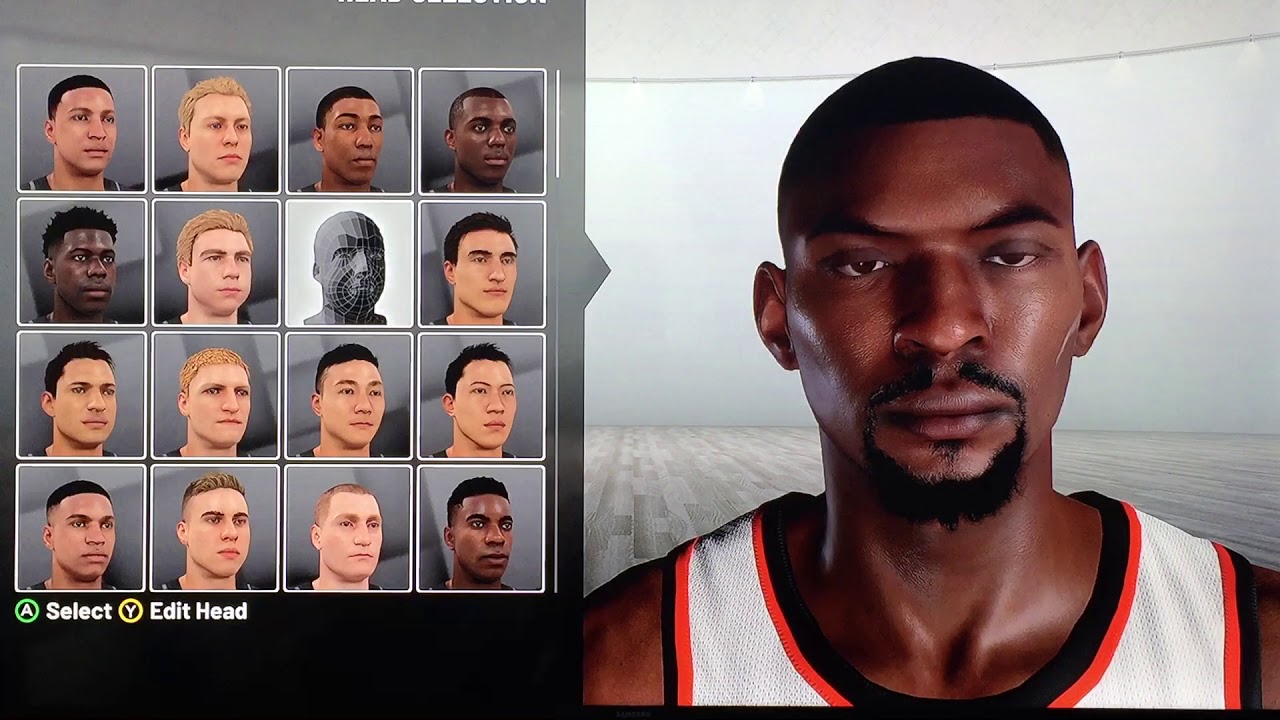In the photo, a diverse group of individuals is depicted with various hairstyles and appearances. The group includes:

- A guy with short black hair.
- Another guy with short black hair.
- Two white guys with blonde hair.
- Several black guys with short black hair.
- One white guy with short blonde hair.
- A white guy with nearly bald hair.
- An Asian individual with short black hair.
- A half-black guy with short black hair.
- A white individual with frosted short hair.
- A Mexican individual with short black hair.
- A black guy with somewhat short hair on the left side of the image.

In the center of the image, there is a notable interface with the word "A" in green, "Select" in white, and "Y" in yellow, along with the words "Edit Head" in white. 

On the right side of the image, there is a black guy with short black hair wearing a white tank top. His eyes appear slightly droopy and cross-eyed, giving the impression that he may have suffered a head injury at some point, resulting in a perpetually vacant or confused expression.

The background consists of a white room with a gray, tiled floor.